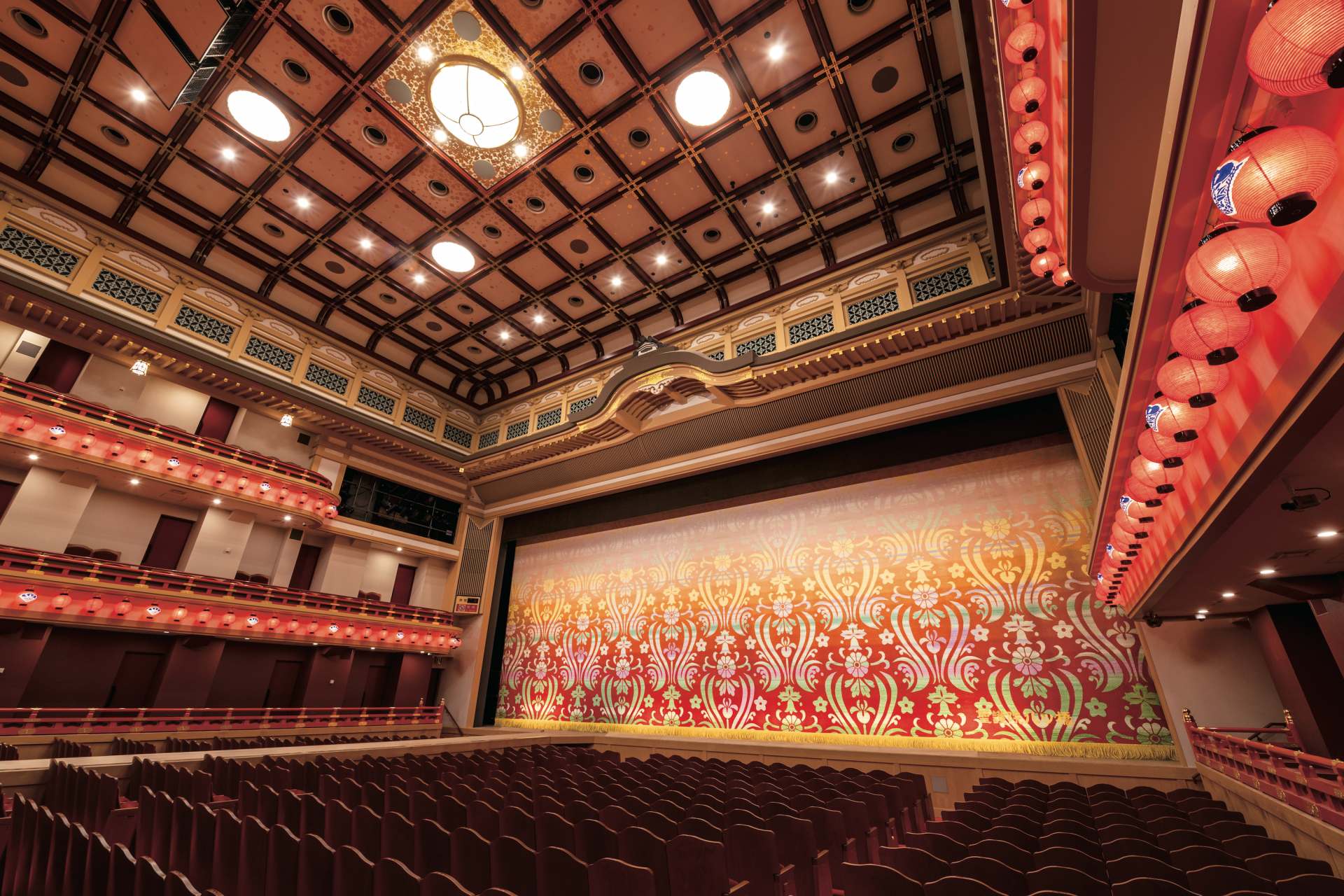This is an intricate and expansive performance theater captured from an unusual angle. The viewpoint is from the right side, towards the back and lower end of the auditorium, revealing an elaborate multi-tiered seating arrangement. The seats are mostly wooden and closely connected, extending towards the stage in the center. An aisle runs beside these seats, leading to a larger middle section and another aisle beyond, flanked by more seating barely visible on the left.

The bottom level is distinct with rows of seats, followed by an ascending layout of balconies. Each balcony features a front row adorned with red Chinese paper lanterns. In the midsection of the theater, railings and doors are aligned vertically, with additional seating on the second level. Above this, a glass-encased booth is situated close to the stage, contributing to a meticulously designed viewing arrangement.

The stage itself is modest in depth but vividly decorated with a red curtain adorned with white symbols and a flowery pattern of green, pink, yellow, and white. Above the stage, the roof is a tapestry of decorations, lights, and grids. Rounded orange lights and black rectangles with white spots pepper the ceiling and walls, giving an opulent and somewhat whimsical feel to the theater. The ceiling is exceptionally high, adorned with ornate, unnecessary detailing, contributing to the grandeur.

The image, in landscape orientation, shows an entirely empty, well-lit theater, seemingly prepped for an evening show. The absence of people emphasizes the vastness and intricate beauty of the structure, evoking a sense of awe and wonder at its design reminiscent of old-world theaters.